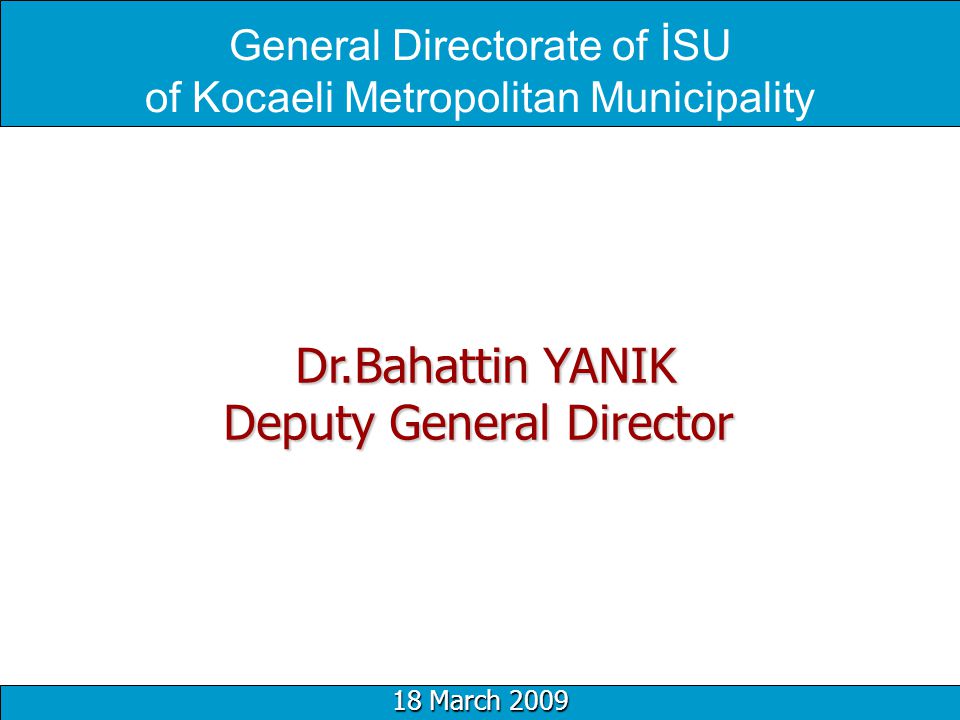This single slide from a larger presentation is divided into three sections. The top section features a thin blue banner with white text that reads, "General Directorate of ISU of Coquille Metropolitan Municipality." The central section, which is the largest, has a white background with prominent red text displaying, "Dr. Bahattin Yanik, Deputy General Director." Both "Bahattin" and "Yanik" are spelled as B-A-H-A-T-T-I-N and Y-A-N-I-K, respectively. The bottom section, a thin blue banner, mirrors the top banner’s color and contains white text that marks the date "18 March 2009." This composition presents a structured and clear visual layout typical of a formal presentation slide.